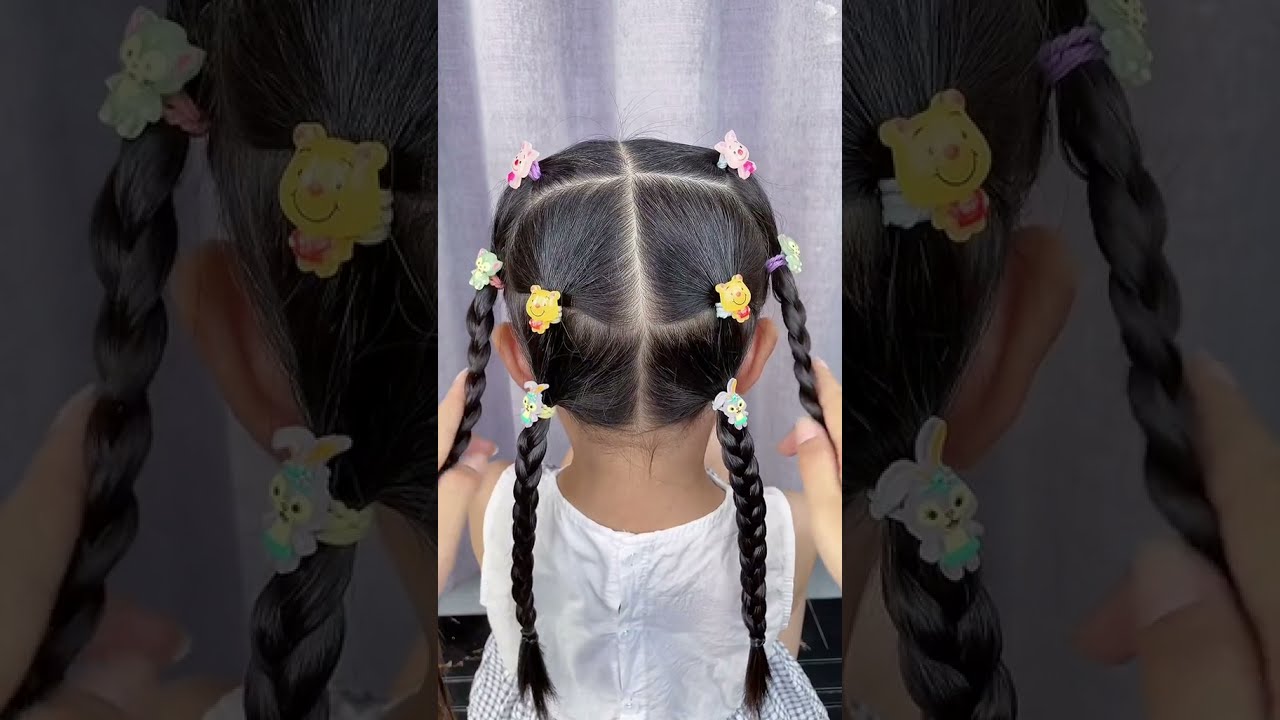An intricate image depicts the back of a young girl's head, her dark brown to black hair meticulously styled into four distinct braids. She wears a pristine white dress, visible from the waist up, and her fair skin contrasts with her dark hair. Various character-themed barrettes adorn her hair, including seven notable clips that feature a mix of beloved figures: two yellow Winnie the Pooh bears with red shirts, two gray bunnies, a purple bunny with a green skirt and green flower, and two pink bears resembling Piglet. The scene captures a supportive moment as a woman's hands are seen carefully holding the girl's braids, possibly adjusting or fixing them. The image itself is creatively framed within two larger but darker and more zoomed-in versions of the same picture, adding a layered depth to the photograph.